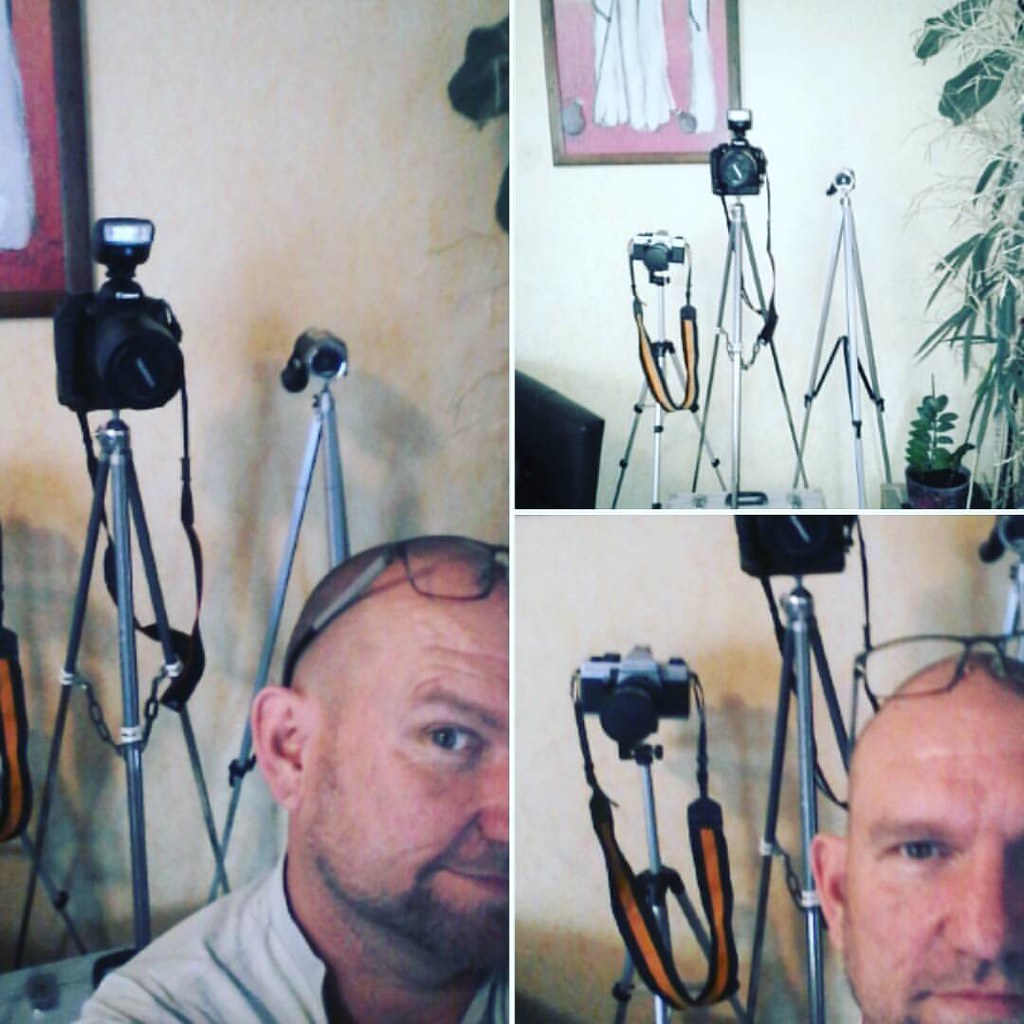The image is a composite of three related photographs, showcasing multiple angles of the same scene. On the left, a vertically oriented rectangular photograph occupies the space halfway into the middle. Here, a man with glasses resting on top of his head is seen, though only one eye and half of his face are visible, giving a partial view including his ear. This left-side image depicts two cameras on tripods pointed at the photographer.

To the right, the space is divided into two smaller photographs stacked vertically. The top photograph captures three cameras, all on tripods, aimed towards the photographer with a wall backdrop and a hint of a pink picture featuring white figures. The bottom right photograph shows the same man from the left image, again with glasses perched on his head, and a very slight smile. However, his face is still partially obscured, and all three cameras on tripods are visible in the background, though the far right camera is barely discernible.

The three images together provide a detailed multi-perspective view of a scene involving a man and several tripoded cameras.